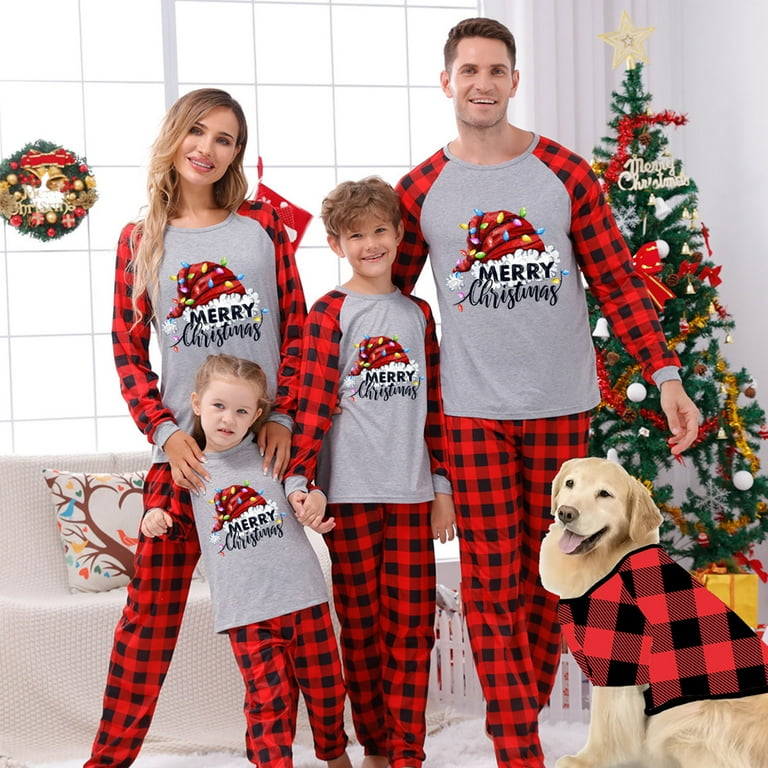The image captures a festive family portrait featuring parents, their two children, and their golden retriever, all dressed in matching Christmas pajamas. The pajamas are characterized by red and black buffalo plaid sleeves and pants, while the body is gray and adorned with a Santa hat wrapped in colorful Christmas lights and the words "Merry Christmas." They are positioned before a white backdrop, which includes a white couch, a decorated Christmas tree with a gold metal star on top, and a wreath hanging in the window. From left to right, the young mother holds her daughter, who leans back into her, while the son stands in the middle. The father stands to their right, with an arm around the son, and the family's golden retriever, also donning a matching plaid outfit, sits at the father's feet on the far right. The dog seems slightly out of place, as if digitally added to the scene.